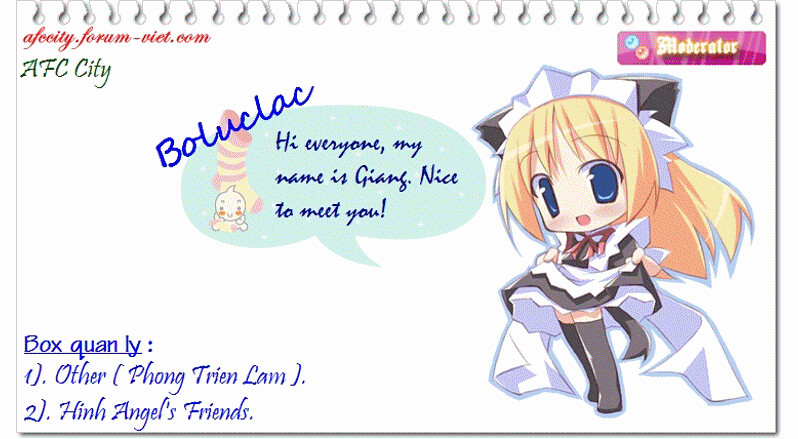The image depicts a horizontally positioned, cartoonish piece of paper appearing to have been ripped out of a spiral notebook. On the right side, there's an anime-style maid with long blonde hair tied in an up ponytail, blue eyes, and wearing a traditional black and white maid outfit complete with knee-high socks or boots and a white bandana on her head. A red bow accentuates her neckline. The character is holding up her skirt modestly. In the center of the page, a speech bubble from the maid says, "Hi everyone, my name is Gene. Nice to meet you." Inside this speech bubble, there is a red stocking and a faded, childish-looking figure. The top left corner holds an indecipherable cursive website address, seemingly afccity.forum.com, and the letters "AFCCITY" appear again at the bottom. The bottom left has somewhat hard-to-read, blue font text that says "BOXPLANLY, one other fawn tree and lamb, and then two pin angels friends." The overall paper conveys a mix of organized text and whimsical animated artwork.